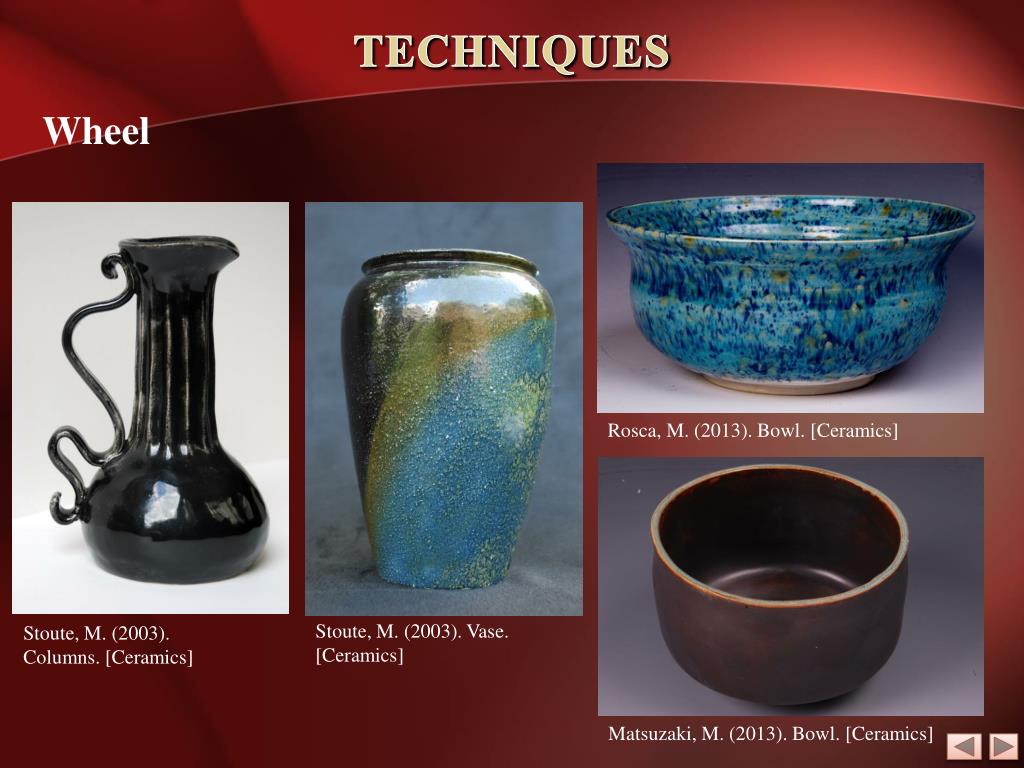This image appears to be a page from a textbook or art gallery book featuring ceramic techniques. The background of the page is a rich, gradient red. The top section of the page is labeled "Techniques" in British spelling, with the word "Wheel" in white text at the bottom left.

On the far left, there's a 2003 ceramic column piece by Stout M. It has a white background and a black vase with a rounded bottom, a cylindrical top, and a swirly handle reminiscent of a hookah.

The central image showcases another Stout M 2003 creation. This vase features a gradient of blue, yellow, and black, embedded with white dots and a smooth, glossy surface. It gives the impression of being suitable for holding umbrellas or canes due to its stature and decorative quality.

To the upper right, the page displays a blue ceramic bowl by Rosca M from 2003. The bowl is light blue with dark blue and orange speckles, featuring a wide rim and squat shape.

Below this, there is another ceramic bowl from 2003 by Mitsuzaki M. This brown bowl has a wooden-like appearance and closely resembles a small rice bowl, with a simple and understated design.

Each piece is meticulously detailed in the images, highlighted against the striking burgundy-red background of the page.